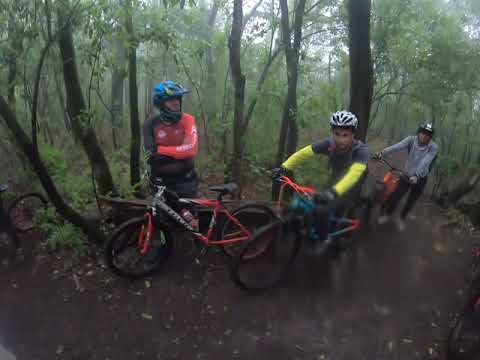In a dense forest shrouded with fog and dim light from a gray sky, three young dirt bikers have paused their ride on a narrow, barely visible dirt trail. The forest around them is thick, with tall tree trunks close by and leafy canopies higher up. The biker at the forefront, wearing a teal helmet and a red shirt, stands beside his red and black dirt bike, possibly signaling a break. Ahead of him, another rider in a gray t-shirt with yellow sleeves and a silver helmet sits astride his bike, looking back at the others. The third biker, donned in a gray sweatshirt and black pants, walks his bike with a red frame and a black helmet, trailing slightly behind the group. The scene captures the nuances of a quiet moment in nature, framed by the lush greenery and the intricate interplay of light and shadow in the forest.